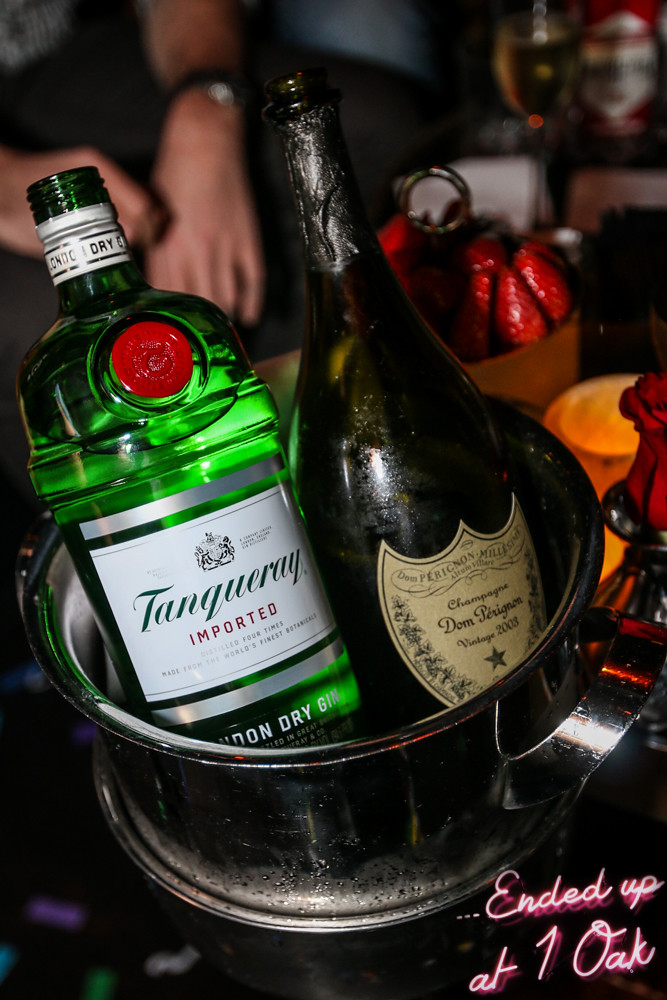This color photograph captures a close-up scene on a table, dominated by a large, brightly lit silver champagne bucket. Inside, there is a bottle of Dom Pérignon Champagne, potentially vintage 2001, 2003, or 2009, nestled beside a green bottle of Tanqueray London Dry Gin with its signature white label and red seal. The ice bucket, covered in condensation, reflects the ambient light, enhancing its metallic sheen. In the background, the image reveals blurred, intimate lighting with yellow-orange hues and partially visible food items, possibly including red chicken wings or strawberries. A person's forearms and hands with a wristband or watch subtly frame the scene from behind. In the bottom right corner, the text "ended up at One Oak" is illuminated in neon white and pink, suggesting a vibrant setting, likely in a club or bar.